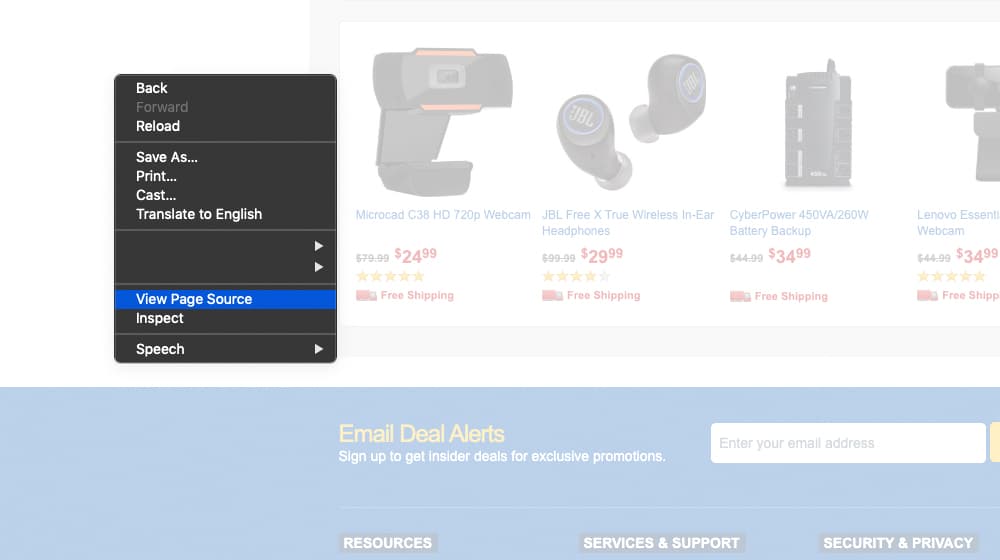A partially transparent screenshot of an online store page displays four products in a row: a webcam, Bluetooth headphones, a battery, and a blue webcam. Each product listing includes an image, a blue hyperlink with the product name, a price in red, a store rating, and a "free shipping" note. On the left side of the screenshot, a dark gray right-click menu typical of Windows operating systems appears, featuring white text options such as "Back," "Forward," "Reload," "Save as," "Print," "Cast," "Translate to English," "View page source," and "Inspect." The "View page source" option is highlighted in blue, indicating it's currently selected.